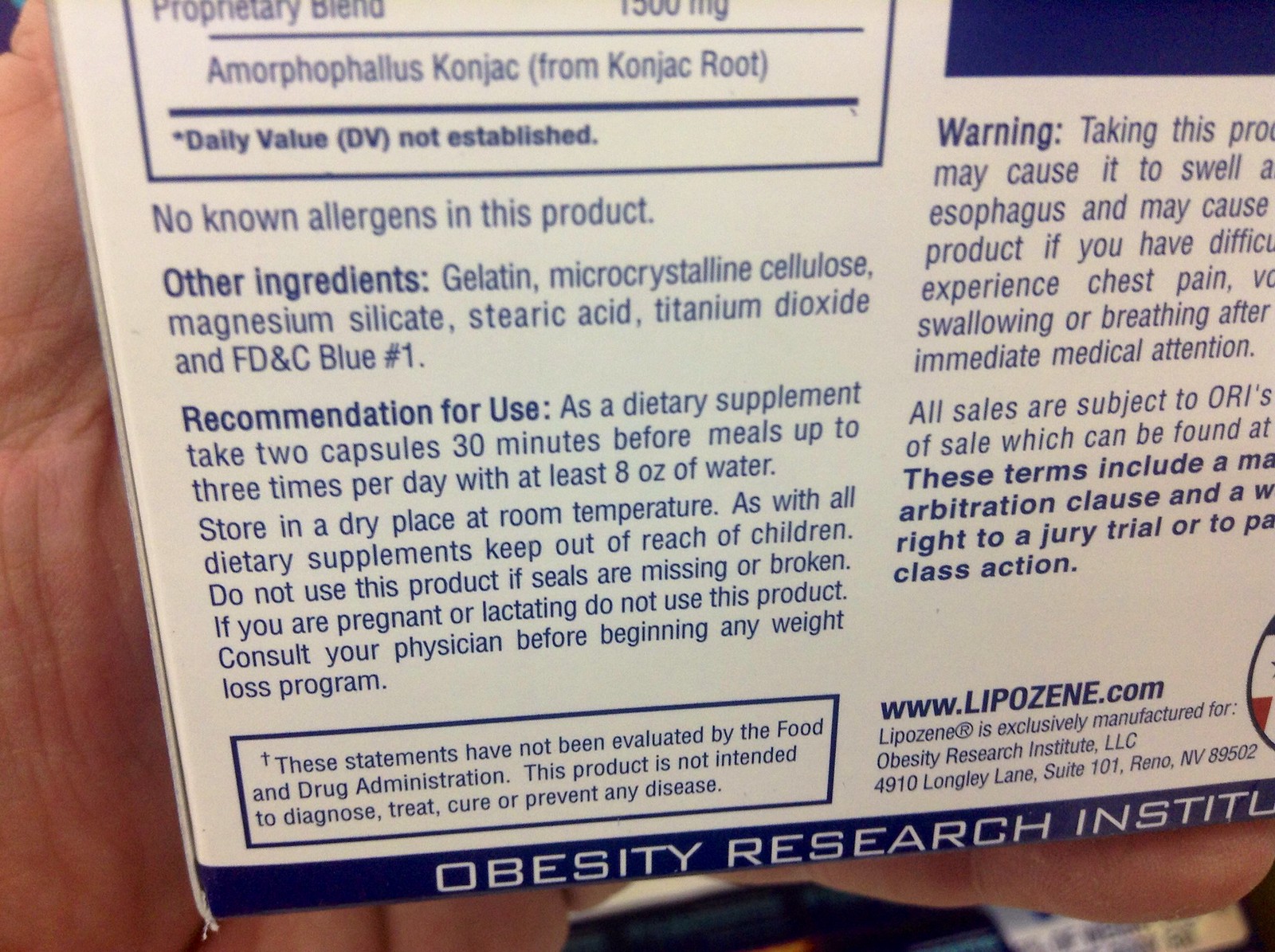In this image, a hand with light skin is holding a retail box, with the rest of the person cropped out beyond the middle of their hand. The box is predominantly white with a distinct blue border along the bottom edge. Displayed in white letters on the blue border is partially visible text reading, "Obesity Research In," which likely continues to say "Institute." The forefront of the box contains detailed information about ingredients; however, only the "other known ingredients" are visible, as the active ingredients are cropped out at the top of the image. Additional details such as usage recommendations and warnings are present, though these too are partially obscured. The box features a website, www.lipozene.com, which is associated with the product being promoted within the box.